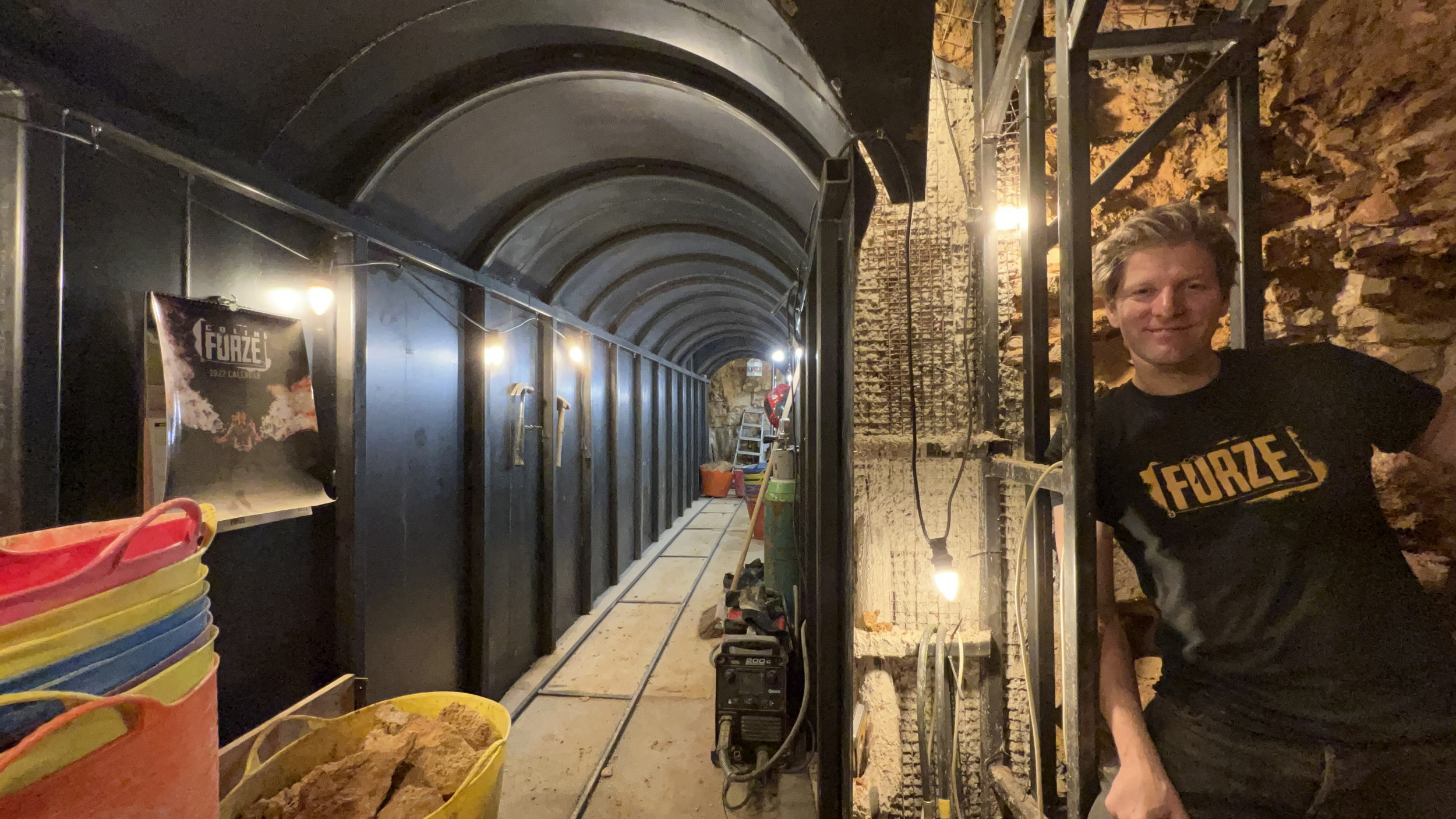The photograph depicts a man with short, windswept blonde hair, standing and smiling to the right side of the frame within a tunnel. He is leaning against a metal support structure, with lights hanging intermittently from visible cables, illuminating the rocky, hewn walls of the cave behind him. The man, who is white, is dressed in a black t-shirt with yellow text spelling "FURZE." The tunnel itself appears to be a hybrid space combining elements of mining and possibly subway construction. To the left side of the image, there is a structured and ribbed metal archway, lined with beams and metal panels, leading further into the tunnel. The foreground is cluttered with yellow, blue, and orange plastic totes, some of which are filled with rocks, suggesting ongoing excavation activities. Various tools, like mop buckets, brooms, machinery, a ladder, and mining implements such as hammers or pickaxes, are scattered around the area, highlighting its industrial use. The scene is further characterized by rail tracks running along the tunnel floor and a poster with the text "FURZE."